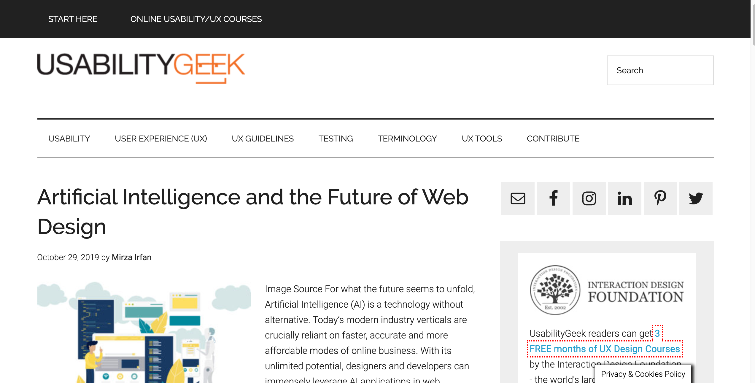This screenshot captures the homepage of a website called Usability Geek. In the upper left corner, there is a black header containing a link labeled "Start Here" in white font. To its right, there is another link that reads "Online Usability/UX Courses." Below this header, the website's title and logo, "Usability Geek," are prominently displayed; "Usability" is in black, and "Geek" is in orange, both in all-capital letters. Adjacent to the logo on the far right is a search bar.

Beneath this title row lies a navigation menu with several items listed: Usability, User Experience (UX), UX Guidelines, Testing, Terminology, UX Tools, and Contribute. Directly below this navigation menu, the title of the featured web page, "Artificial Intelligence and the Future of Web Design," is displayed. To the right of the title, there are various social media sharing icons. 

The body of the page begins with the publication date, "October 29th, 2019," and the author's name, "by Mirza Irlan." Below this, a vector image is positioned alongside a brief description and some introductory content about the topic of the page.